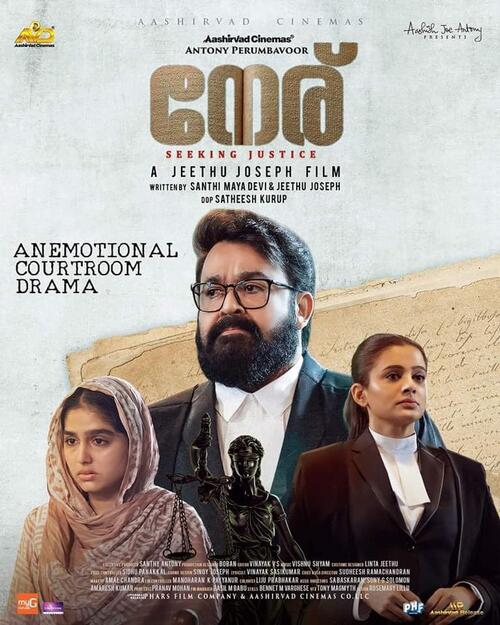The image is a brightly lit, clear movie poster for the film "Seeking Justice," an Ajithu Joseph production presented by Asher Vahd Cinemas and Antoni Perumbavvor. The poster features a grayish and cream-colored background, with prominent text at the top reading "Asher Vahd Cinemas." The header also mentions "Goda Seeking Justice" and "a Jesu Joseph film." 

Beneath this, the main characters are displayed and prominently centered is a man with brown hair, a full black beard, and glasses. He is dressed formally in a black tuxedo with a white undershirt and tie. Beside him stands a woman in a business-styled jacket with a white blouse, her long brown hair pulled back in a ponytail, and a strap over her shoulder hinting at a purse. On the other side stands a Muslim woman in a traditional shawl covering her hair and draped over her shoulder. A black statue holding weights is also visible, adding to the courtroom theme. Above the trio, text reads "An Emotional Courtroom Drama," indicating the film's genre. Additional writing appears below, further detailing the film.